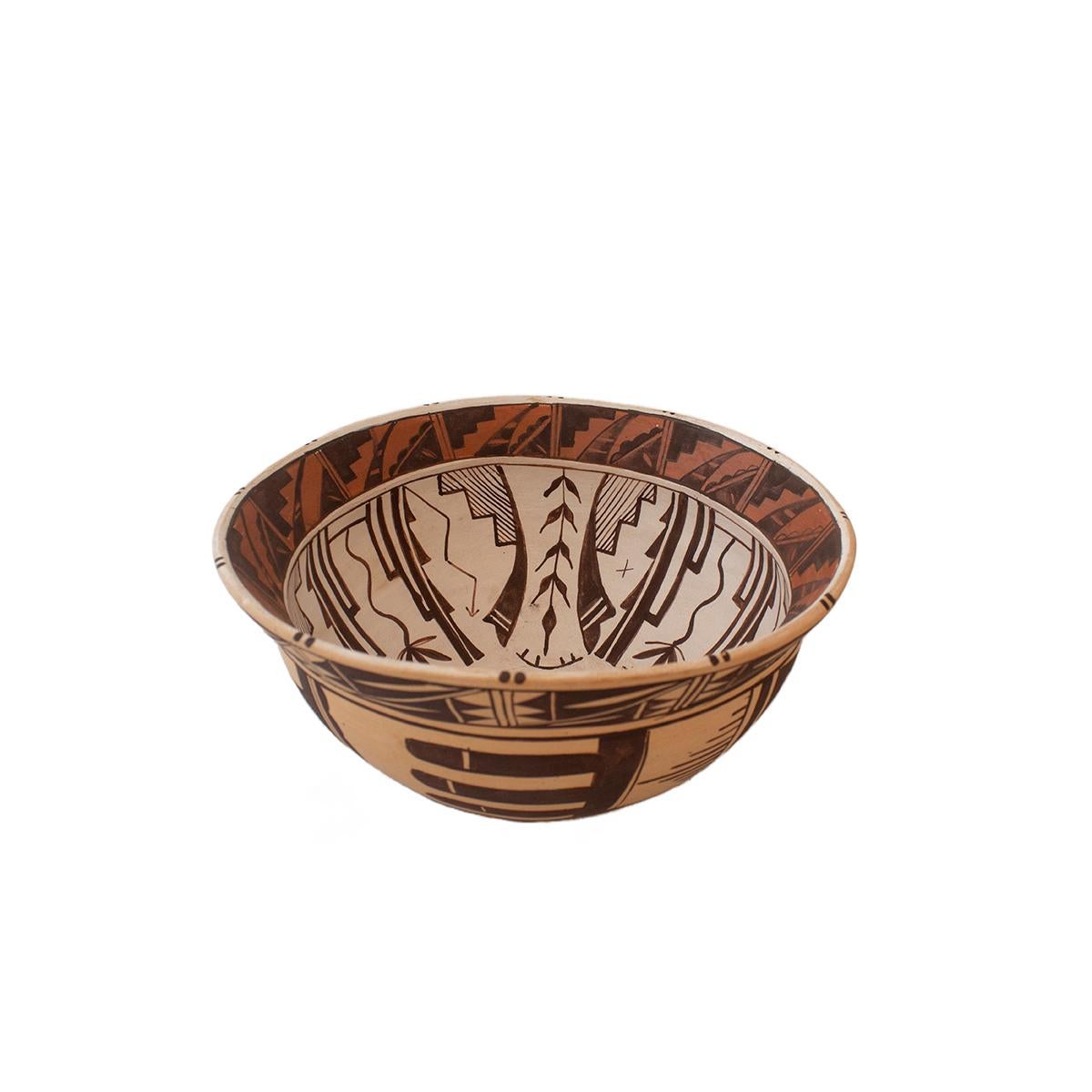The image is a color photograph in a square format, featuring a handmade bowl that appears to be made of either wood or ceramic. The bowl is predominantly decorated in shades of brown, black, orange, and tan. The background is entirely white, giving the impression that the bowl floats in space.

The outside lip of the bowl is a tan color, adorned with geometric patterns made up of orange lines against a black background, which form shapes similar to the letter 'N' encircling the bowl. This pattern extends around an inch in height from the lip.

Inside the bowl, the rim is golden, decorated with a repeating pattern of brick red and black geometric shapes. The central area of the bowl features intricate dark brown or black designs on a tan background, including elements such as leaves, arrows with wing-like attachments, palm trees, and buildings. These illustrations are detailed and create a high-contrast, linear aesthetic that suggests Photographic Representationalism Realism. The overall presentation of the bowl highlights both its artistic craftsmanship and the complexity of its decorative motifs.